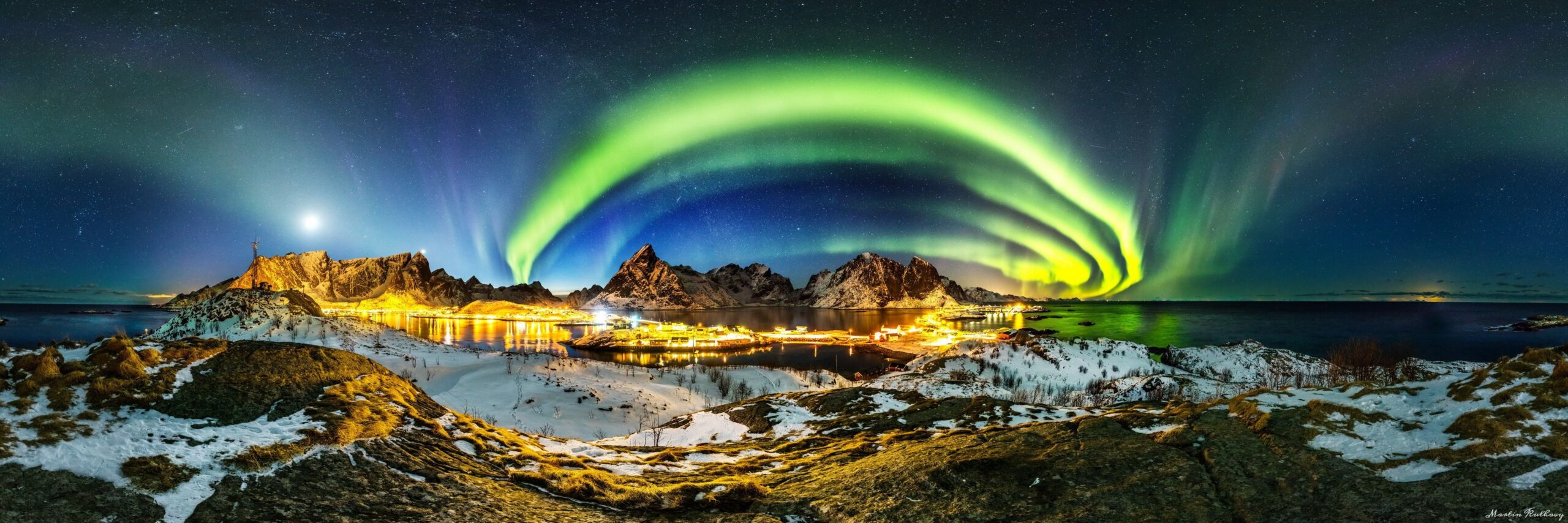In this vivid panorama shot of a nighttime landscape, the serene beauty of the Northern Lights (Aurora Borealis) takes center stage with its mystical green and purple hues, casting a magical glow over the entire scene. The foreground reveals a snowy ground leading to a calm lake, surrounded by majestic mountains dusted with snow. The night sky is awash with a myriad of stars, and to the left, a bright, white moon illuminates the landscape. In the distance, a city or town sparkles with golden and white lights, perhaps enhanced by the ethereal glow of the Northern Lights. The scene is almost surreal, blending natural wonders with hints of urban illumination, all under the dome of an enchanting star-filled sky.